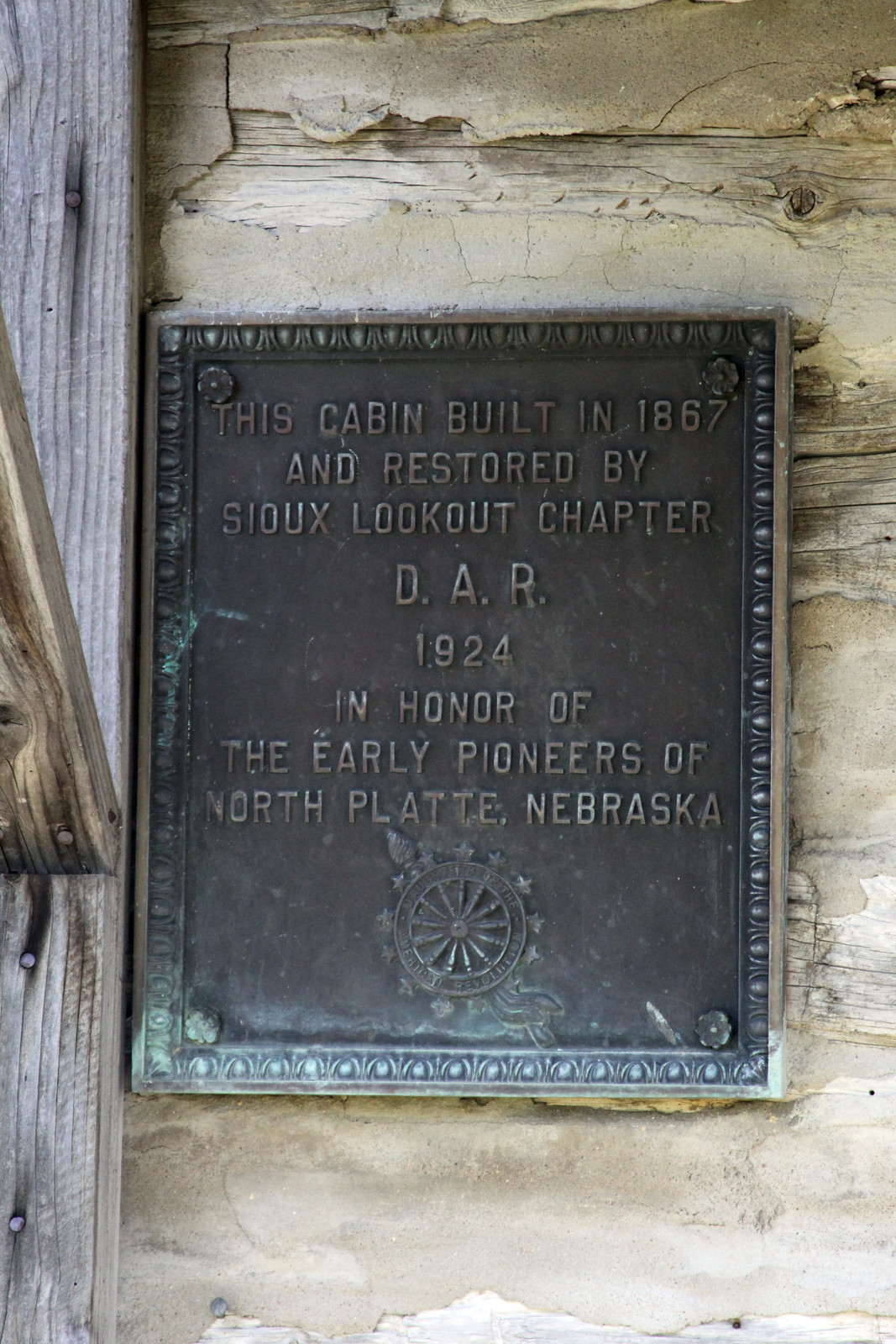This photograph showcases a tall, rectangular metal sign affixed to an aged wooden wall. The sign, rendered in a dark gray or almost black metal with noticeable green oxidation, is framed and bolted at each corner with bolts resembling tiny flowers. The text on the sign reads, "This cabin built in 1867 and restored by Sue's Lookout Chapter DAR 1924 in honor of the early pioneers of North Platte, Nebraska." Below the text, there is an engraving of a wheel adorned with stars around its edges and a ribbon extending from the bottom. The background wall comprises light tan, chipped wooden logs that appear to have been covered with plaster now cracked and revealing the wood beneath. Additionally, to the left of the sign, a tall gray wooden plank, embedded with nails, stands out against the aged, light brown and gray tones of the wooden wall.